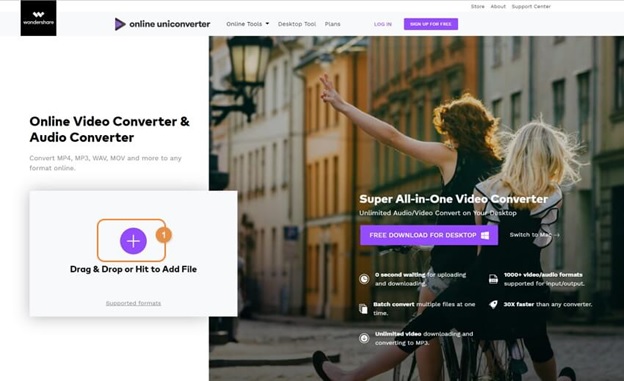The web page appears to be for an online media conversion service, possibly named "W" based on the black square logo with a white "W" in the upper left-hand corner. Accompanying this logo is some white text that is too small to discern clearly. Adjacent to the logo is a right-pointing triangle with a black border and a purple interior, directing attention to the text "Online Uni Converter." 

Further along the top navigation bar, there are several options: "Online Tools" with a drop-down menu, "Desktop Tools," "Plans," a "Login" button, and a prominently featured purple "Sign Up for Free" button. Below the company logo and main navigation, bold text reads "Online Video Converter and Audio Converter," advertising the capability to convert various formats such as MP4, MP3, WAV, MOV, and more to any desired format online. 

Directly beneath this introductory text, there is a user interface element designed for file uploads, indicating users can drag and drop files or click to add them, with supported formats listed nearby. 

Occupying the middle to right section of the page is an engaging image depicting two women riding bicycles, seemingly through a vibrant New York City scene, viewed from behind. Overlaying this image is text proclaiming "Super All-in-One Video Converter," alongside options to "Download for Free" and "Download for Desktop." Smaller, additional text is present but not legible.